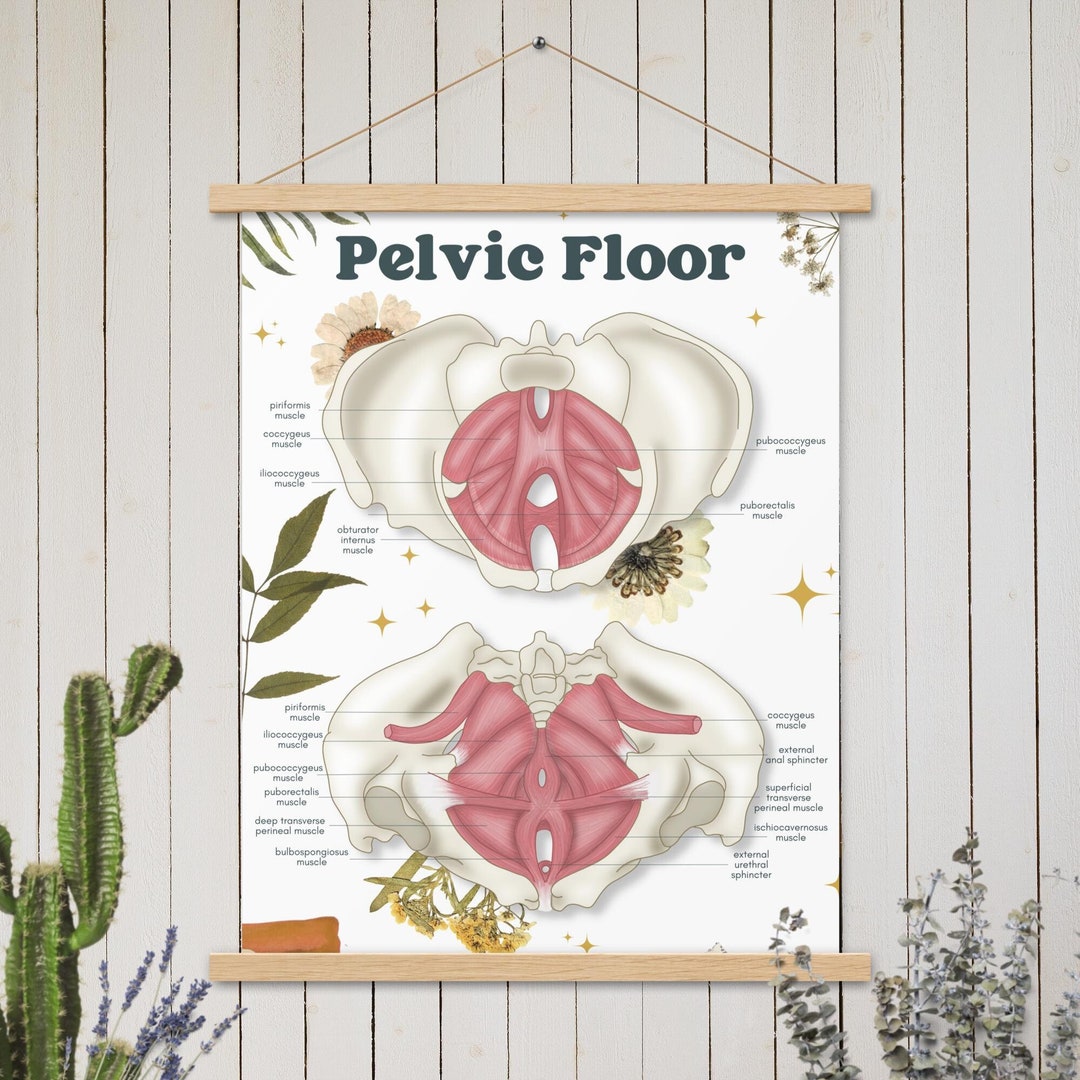This photograph showcases a detailed anatomical diagram of the pelvic floor, displayed as a wall hanging on a striped white-paneled wall. To the left of the hanging, a green cactus with two arms grows from its base, and a nearby blue, grassy flower adds a touch of color. On the right side, a bush with long, thin stalks adorned with small green leaves completes the natural setting. The wall hanging itself is secured by a wood frame and string, and appears to be printed on canvas. The text at the top of the canvas reads "Pelvic Floor," and features two illustrative cross-sections of the pelvis, demonstrating both bone mass and muscle structures. The diagram encompasses labeled muscles including the piriformis, coccygeus, iliococcygeus, obturator internus, puborectalis, pubococcygeus, and others such as the deep transverse perineal muscle, bulbospongiosus muscle, external anal sphincter, superficial transverse perineal muscle, and the ischiocavernosus muscle, as well as the external urethral sphincter. The illustrations, while not entirely realistic, are highly detailed and informative.